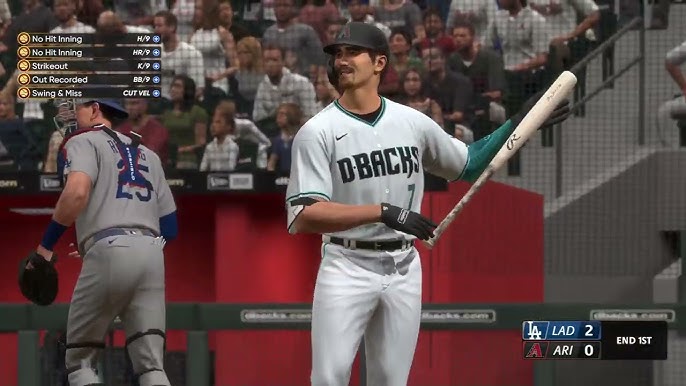This image, likely a screenshot from a baseball video game, portrays a detailed scene from a game between the LA Dodgers and the Arizona Diamondbacks. In the foreground, a Diamondbacks player, dressed in an all-white uniform with black writing and a black helmet, is standing at the plate, gazing out to the left. Behind him, the catcher, clad in a different uniform, is in motion, with his back facing the audience. Above the players, various game statistics are displayed, including "no hit inning," "strikeout," "out recorded," and "swing and miss." The top-left corner features detailed stats, possibly tracking game achievements. The background showcases an audience seated in the stands, bordered by a red wall and gray steps, with a gate separating them from the field. In the bottom right corner, the score is visible, reading "LAD 2, ARI 0" at the end of the first inning.